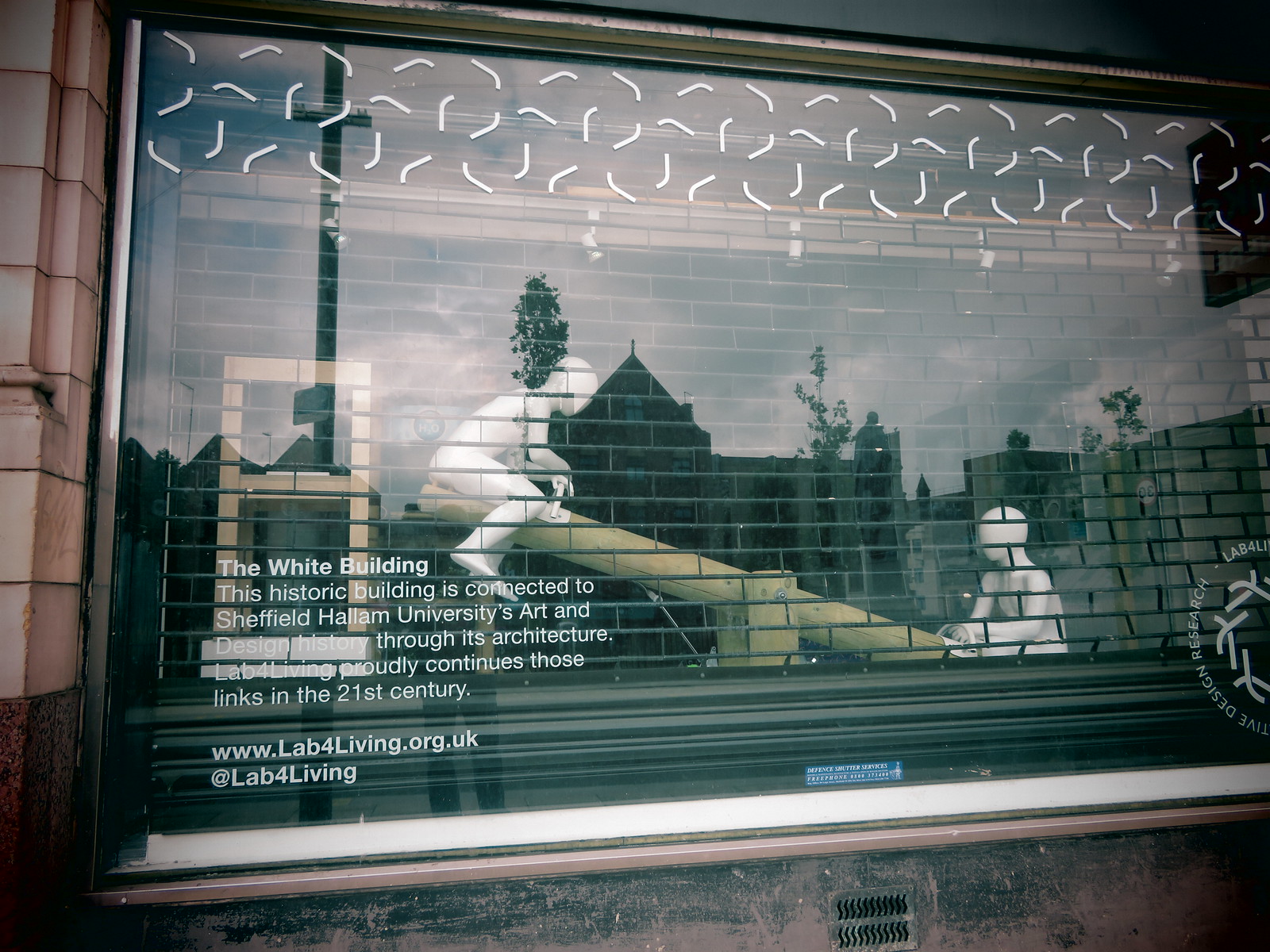This image depicts a storefront window featuring a chain link security gate on the inside, behind which are two white child mannequins positioned on a wooden seesaw. The mannequin on the left is elevated in the air while the one on the right sits grounded. Behind the seesaw, shelving can be seen on the left side. The window itself has text printed in white that reads, "The White Building. This historic building is connected to Sheffield Hallam University's art and design history through its architecture. Lab for Living proudly continues those links in the 21st century. www.labforliving.org.uk @labforliving." Additional details include a Lab for Living logo in the bottom right corner of the window, and another indecipherable blue logo in the center at the bottom.